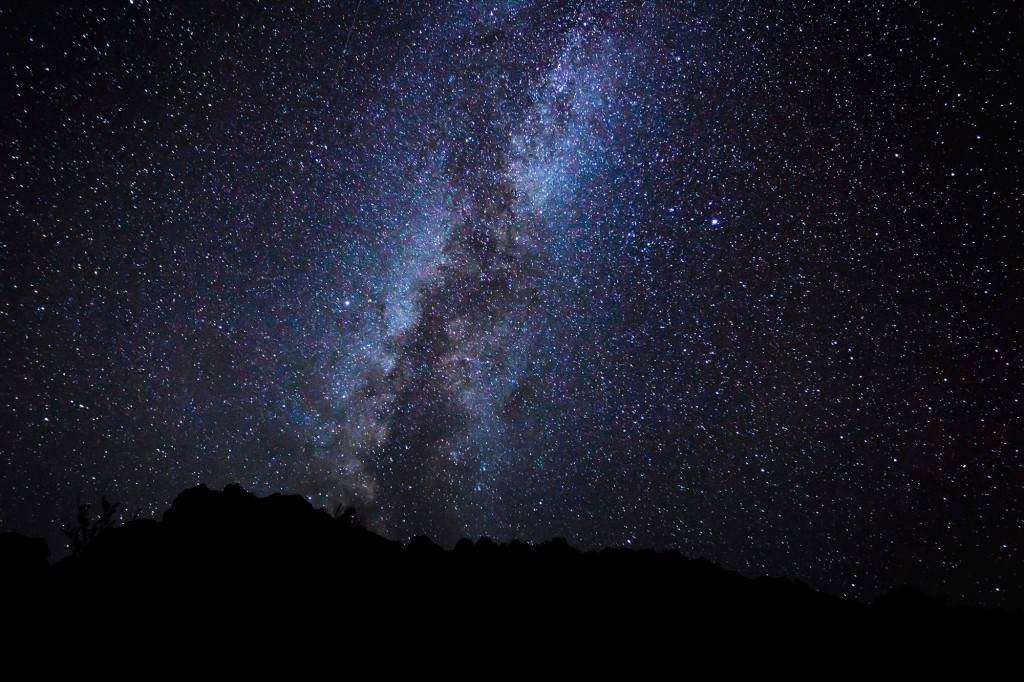In this mesmerizing night sky photograph, the silhouette of a mountain range or foresty area stretches across the bottom, shrouded in an all-encompassing, dark shadow. Above, an infinite expanse of sky is densely populated with millions of stars of various sizes, scattered both closely and distantly from one another. The sky is predominantly black, entirely free from light and regular pollution, allowing the stars to shine brilliantly, more or less uniformly in brightness. Central to the image, a majestic stretch of illuminated cosmic dust in shades of light blue and faint purple runs through, interspersed with darker clouds. This creates a mystical, organic texture devoid of hard edges, giving the scene a soft, luminescent quality. The galaxy's stardust and varied hues—from whites and blues to browns and blacks—enhance the ethereal beauty of this powerful, natural spectacle.